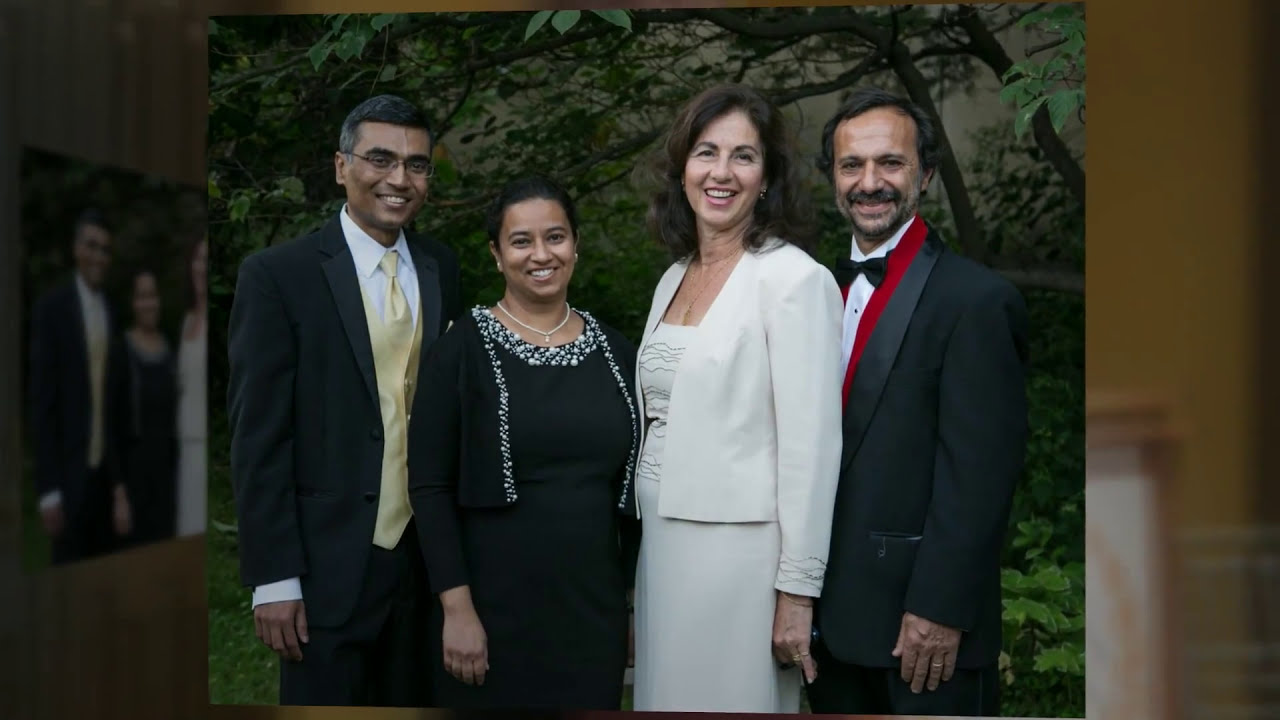In this photograph, four well-dressed individuals are standing side by side, smiling and facing the camera in an outdoor setting. The group is positioned centrally, occupying most of the image, which also features a grassy area, trees, and a building visible in the background. From left to right, the first person is a South Asian man in his 50s, wearing glasses, a black suit, a white shirt, and a yellow tie. Next to him is a South Asian woman in her 40s, dressed in a black dress adorned with white floral lining and wearing a necklace. To her right stands a tall white woman with shoulder-length brunette hair, clad in a white jacket and dress, and exuding a radiant smile. Finally, on the far right is a younger South Asian or mixed-race man with a beard featuring gray streaks, dressed in a black suit, a white shirt, a red vest, and a black bow tie. The photograph captures this elegantly dressed quartet against the backdrop of verdant trees in what appears to be a formal event held outdoors during the day. Vertical rectangular panels framing the left and right edges of the image suggest reflections and nearby furniture elements, possibly indicating a partially mirrored or staged setting, adding depth to the composition.